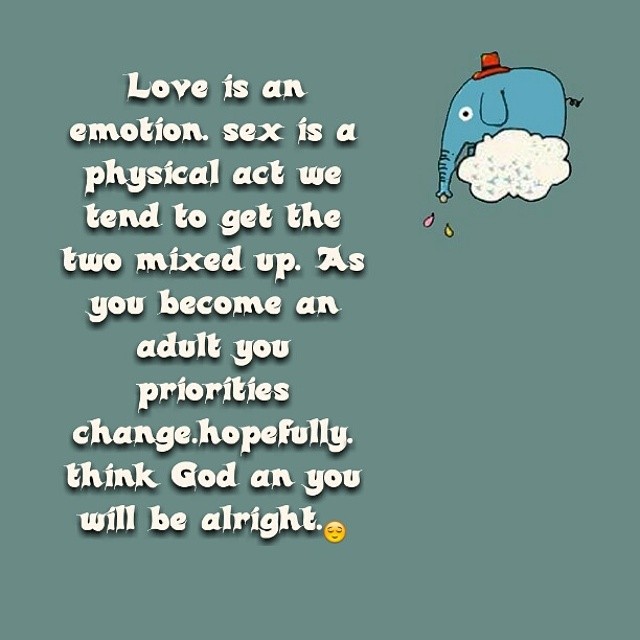The image features a digital, hand-drawn cartoon of a blue elephant, sitting on a white cloud, positioned in the top right corner. The elephant is viewed from a left side profile, wears a red and brown hat, and has a curly tail. Emerging from its trunk are droplets in pink, yellow, and gray, giving the appearance of sneezing. The background is a dark, grayish-green shade. Accompanying the image is white text in a cartoonish block font that reads: "Love is an emotion. Sex is a physical act. We tend to get the two mixed up. As you become an adult, your priorities change, hopefully, thank God, and you will be alright." Positioned towards the bottom center of the image is a yellow smiley face emoji, acting as a period to the text. The style of the image resembles motivational or advisory content often found on social media platforms like Facebook.